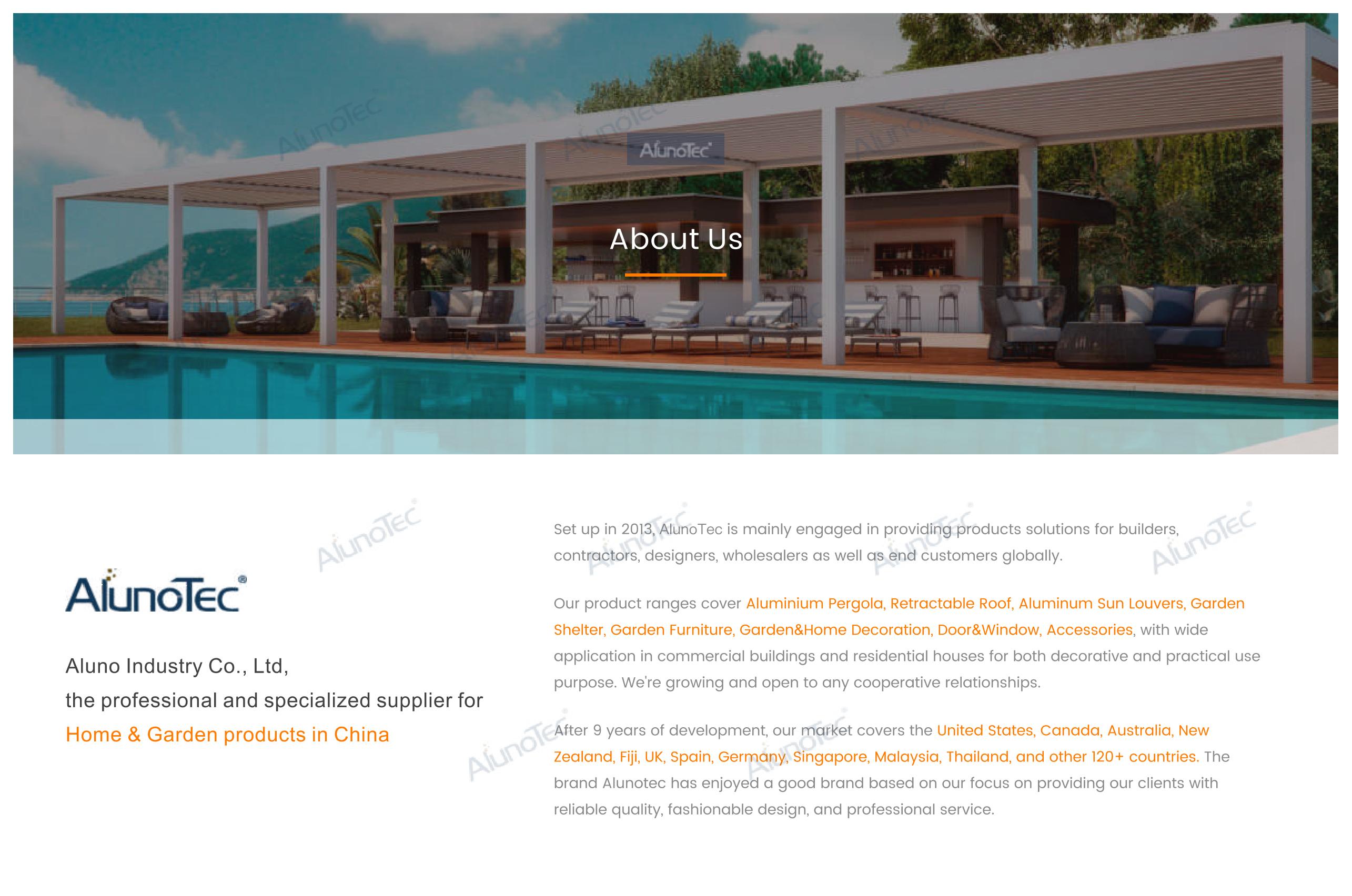A beautiful hero image graces the top of this website, showcasing a serene outdoor area adjacent to a pristine pool, framed by majestic mountains and trees, with an expansive ocean visible in the background under clear blue skies. At the center of the image, the words "About Us" are prominently displayed. The outdoor space features a stylish seating arrangement with numerous chaise lounges shaded under a sleek, modern pergola. In the background, a chic bar area adds a touch of luxury to the setting, suggesting that this might be part of a high-end hotel or resort.

The scene also includes large rattan round chairs and several cushioned seating options, enhancing the comfort and aesthetic appeal of the area. On the left side of the image, the brand name "Alunotech" (A-L-U-N-O-T-E-C) is displayed, with a watermark reading "Aluno Industries Company Limited" at a slight angle across the entire image. This watermark, though somewhat obtrusive, identifies Aluno Industries as a professional and specialized supplier for home and garden products based in China.

A section of text on the right side elaborates on the company's offerings, highlighting their aluminum pergolas, retractable roofs, aluminum sun louvers, garden shelters, furniture, decorations, and accessories. The text also details Aluno Industries' expansion into the U.S., Australia, and various other international markets. Established in 2013, the company primarily provides solutions for builders, contractors, designers, wholesalers, and customers worldwide.